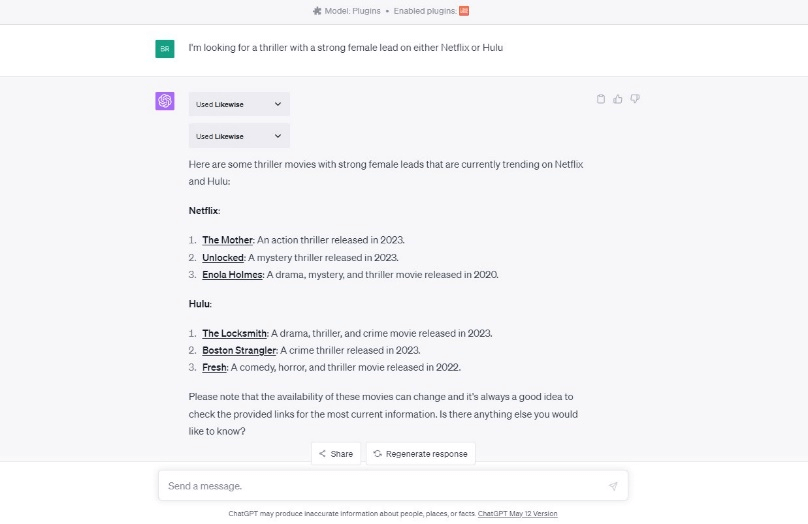This screen capture appears to be from within a somewhat out-of-focus software application, likely a chatbot interface. The predominantly white background is topped by a horizontal gray bar that contains black text reading 'Model Plugins - Enabled Plugins.' On the far right of this bar, there is a red square.

Below the gray bar is a white section featuring a green square, next to which is text that reads, 'I'm looking for a thriller with a strong female lead on either Netflix or Hulu.' Directly underneath this section, within a gray area, lies a purple icon centered with a white spiral. To the right of this icon are two gray drop-down boxes, each with 'Muse' entered as the selection, accompanied by right-pointing arrows.

Further down in this section, the text elaborates, 'Here are some thriller movies with strong female leads that are currently trending on Netflix and Hulu.' Movies available on Netflix are listed in bolded black text as 'The Mother,' 'Unlocked,' and 'Enola Holmes.' Similarly, in bolded black text, Hulu options are listed as 'The Locksmith,' 'Boston Strangler,' and 'Fresh.' The text also notes that availability can change and advises checking provided links for the most current information. 

At the bottom, there are two white buttons labeled 'Share' on the left and 'Regenerate Response' on the right. Below these buttons, a large text entry field displays the placeholder text 'Send message' in light gray. Underneath this entry field, a disclaimer reads, 'ChatGPT may produce inaccurate information about people, places, or faces. ChatGPT May 12th version.'